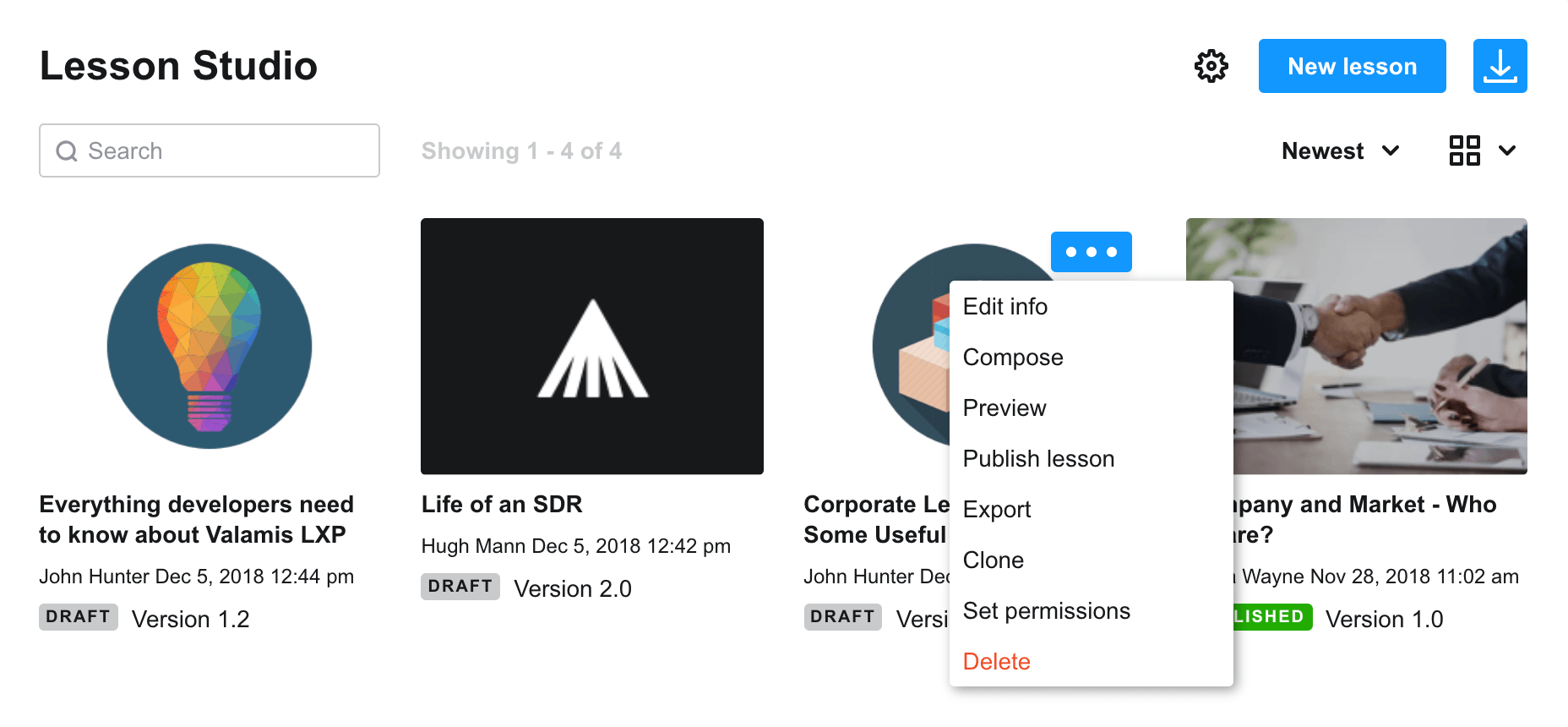Sure, here's a cleaned-up and detailed descriptive caption:

---

Screenshot of the Lesson Studio app.

The interface features a white background. At the top left corner, the app name "Lesson Studio" is displayed in black text. On the top right, there are three buttons: a settings icon, a blue "New Lesson" button with white text, and a blue download icon.

Below these, a small search bar is situated on the left side. Next, there is a label indicating "Showing 1 to 4 of 4". On the extreme right, a toggle labeled "Newest" is visible alongside an icon that allows changing the display layout of the information.

Beneath this toolbar, four search results or lesson entries are displayed:

1. **"Everything Developers Need to Know about Vlamis LXP"** - Accompanied by a multicolored light bulb logo with a green background.
2. **"Life of an SDR"** - Paired with an associated icon.
3. An unreadable lesson title obscured by a dropdown menu offering options including "Edit Info," "Compose," "Preview," "Publish Lesson," "Export," "Clone," "Set Permissions," and "Delete".
4. **"Company and Market"** - Supplemented by an illustrative image explaining the content.

---

This revised caption presents a structured and detailed description of the app's features and layout.